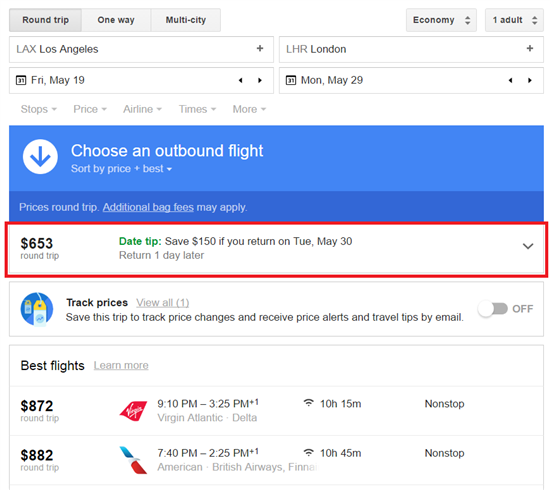The image is a screenshot of a flight booking website. At the top left, there are selectable options in rectangles labeled "Round-trip," "One-way," and "Multi-city." On the top right, a rectangle displays "Economy," with two arrows indicating a dropdown menu, and next to it, another rectangle shows "1 adult" accompanied by up and down arrows for adjusting the number of passengers.

Below these options, there's a white search box where "LAX Los Angeles" is entered as the departure location, and beneath it, "Friday May 19th" as the departure date. To the left, "LHR London" is listed as the destination, with "Monday May 19th" as the return date.

On the left-hand side, in light grey text, there are filters labeled "Stops," "Price," "Airline," "Times," and "More," each accompanied by a downward arrow to indicate expandable sorting options. Just beneath these filters, a blue rectangle with a blue arrow inside a white circle reads "Choose an outbound flight - Sort by price (Best)." Below this rectangle, in slightly darker blue text, it mentions that "Prices are round-trip" and that "Additional bag fees may apply."

Following this, a red rectangle highlights a fare of "$653 round-trip" on the left. In the middle, a green prompt with "Date tip" in white text advises in black text that travelers can "Save $150 if you return on Tuesday, May 30th; return one day later." Below this tip, a blue circle with a white and yellow tag inside encourages users to "Track prices" by saving the trip to receive price alerts and travel tips via email.

Further down, there’s a section labeled "Best flights (Learn more)" featuring two flight options: an $872 round-trip and an $882 round-trip. Both options display a symbol for Virgin, characterized by a red triangle with the word "Virgin" and an airplane wing with blue, white, and red colors.